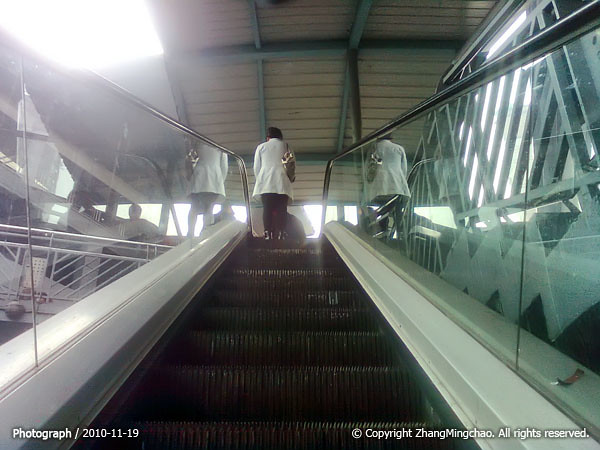This photograph captures a woman riding an escalator that features black steps, white sides, and a clear see-through plastic arm rail with a silver metal top. She is positioned at the top of the escalator, wearing a white jacket over black pants or possibly a long black skirt, paired with black boots. Draped over her right shoulder is a gray or tan handbag. The setting above her reveals a wooden roof overhead, and to the left, faint outlines of people - one seated at a table and another standing - are visible against the bright sunlight, obscuring their faces.